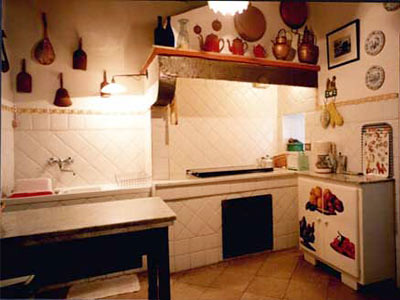This image depicts a quaint, old-fashioned kitchen with a charming, rustic ambiance. The focal point of the space is a small fireplace stove adorned with a shelf above it, showcasing an array of copper pots and tea kettles. The kitchen features a small corner sink with a wall-mounted faucet, while the walls and stove area are lined with shiny white and tan subway tiles. The floor is covered in tan stone tiles, adding to the vintage feel. 

On the right side, there's a distinctive metal cabinet that resembles an old-fashioned refrigerator, its doors decorated with various stickers and images. A kitchen table or island sits in the center, serving as a functional workspace. The walls are adorned with numerous hanging items, including bread spatulas, cutting boards, oven mitts, decorative plates, and a picture frame, contributing to the room's quaint aesthetic. Above the stove, another shelf holds a collection of teapots. The countertops display various kitchen items, emphasizing the room's utilitarian yet cozy vibe.